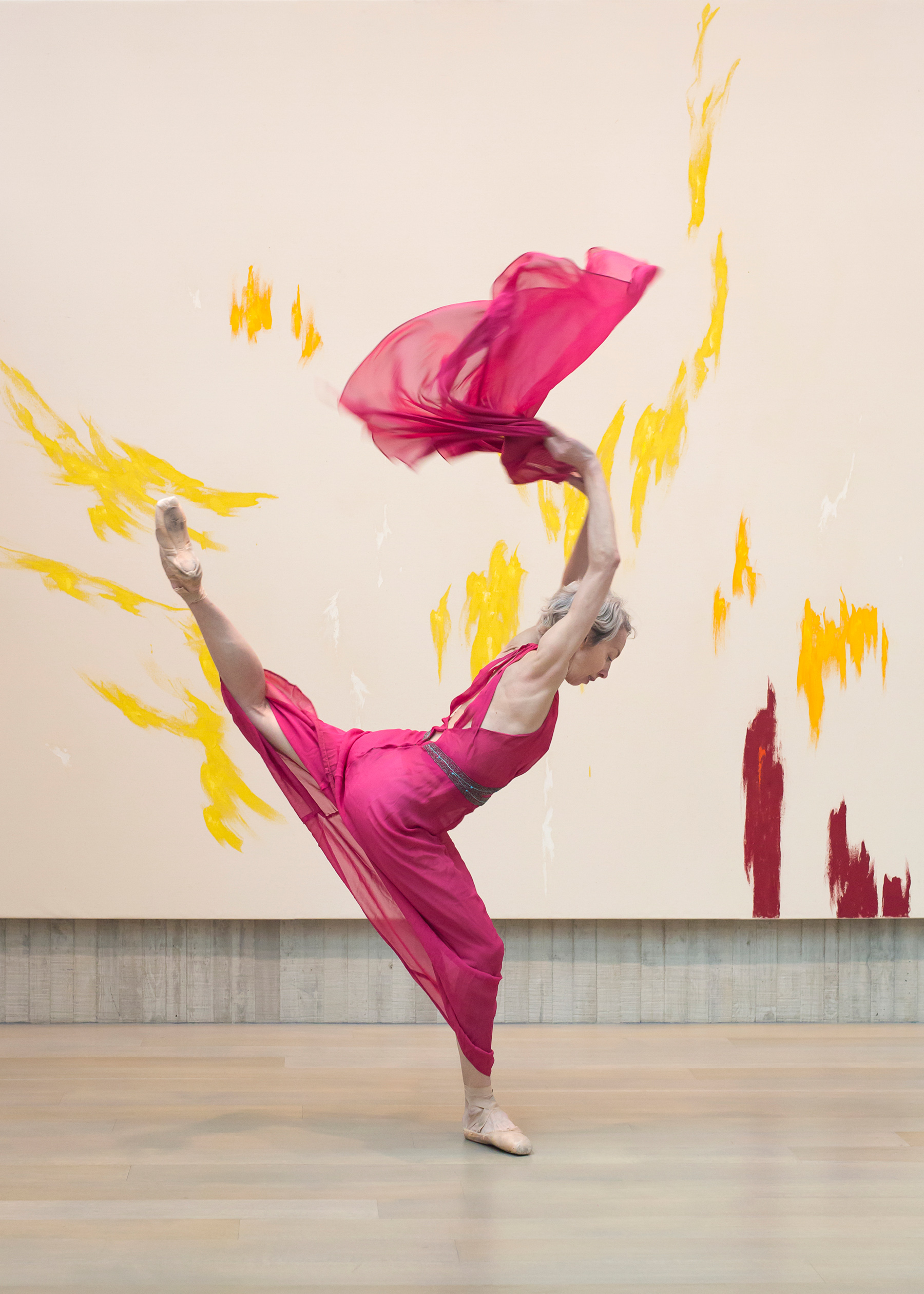The image features a woman dancing on a light hardwood floor, possibly a dance floor. The background resembles an abstract canvas, predominantly off-white with vertical yellow paint lines throughout and a single red vertical line in the bottom right corner. The woman is wearing a purplish-pink outfit with a bit of red in it, complemented by light pink ballet slippers. A sheer, see-through fabric of the same color as her dress drapes from her raised arms, held above her head. Her right foot is planted on the ground while her left leg extends behind her, creating a dynamic split pose. She has a small grayish belt around her waist and her hair appears to be white or silvery, though partially obscured by her arm positioning. The image also shows a bit of wood detail behind her at the bottom, likely part of the floor extending upward slightly. She appears muscular in build, and her head is tilted towards the right, gaze directed downward.